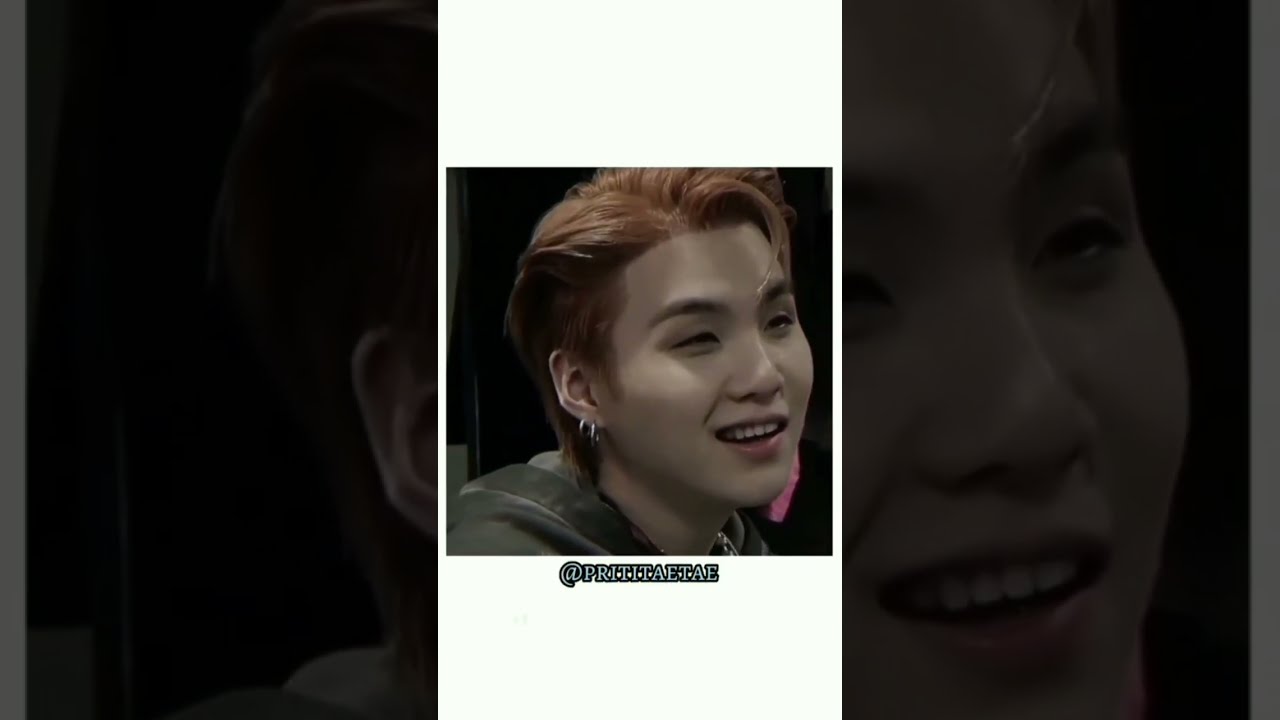This is a highly stylized, AI-created-looking image of an Asian person of indeterminate sex, featuring prominent reddish-auburn, well-groomed, short hair that sweeps upward at the back. The individual is adorned with two hoop earrings made of silver on their earlobes and has perfect, lighter skin. Their gentle and subtle smile adds a sense of warmth as they look upwards toward the top right, as if gazing at something intriguing. They are dressed in a dark gray or black hoodie, with a hint of something pink visible under their chin. The background is a deep black, enhancing the person's striking appearance. The image is centrally framed within a square, bordered by broad white stripes above and below. Additionally, a repeated and enlarged version of the person's face spans the background, lending a surreal quality. At the bottom, there is a social media handle in a bold white font outlined in black, reading "@PREETA_FAYE."